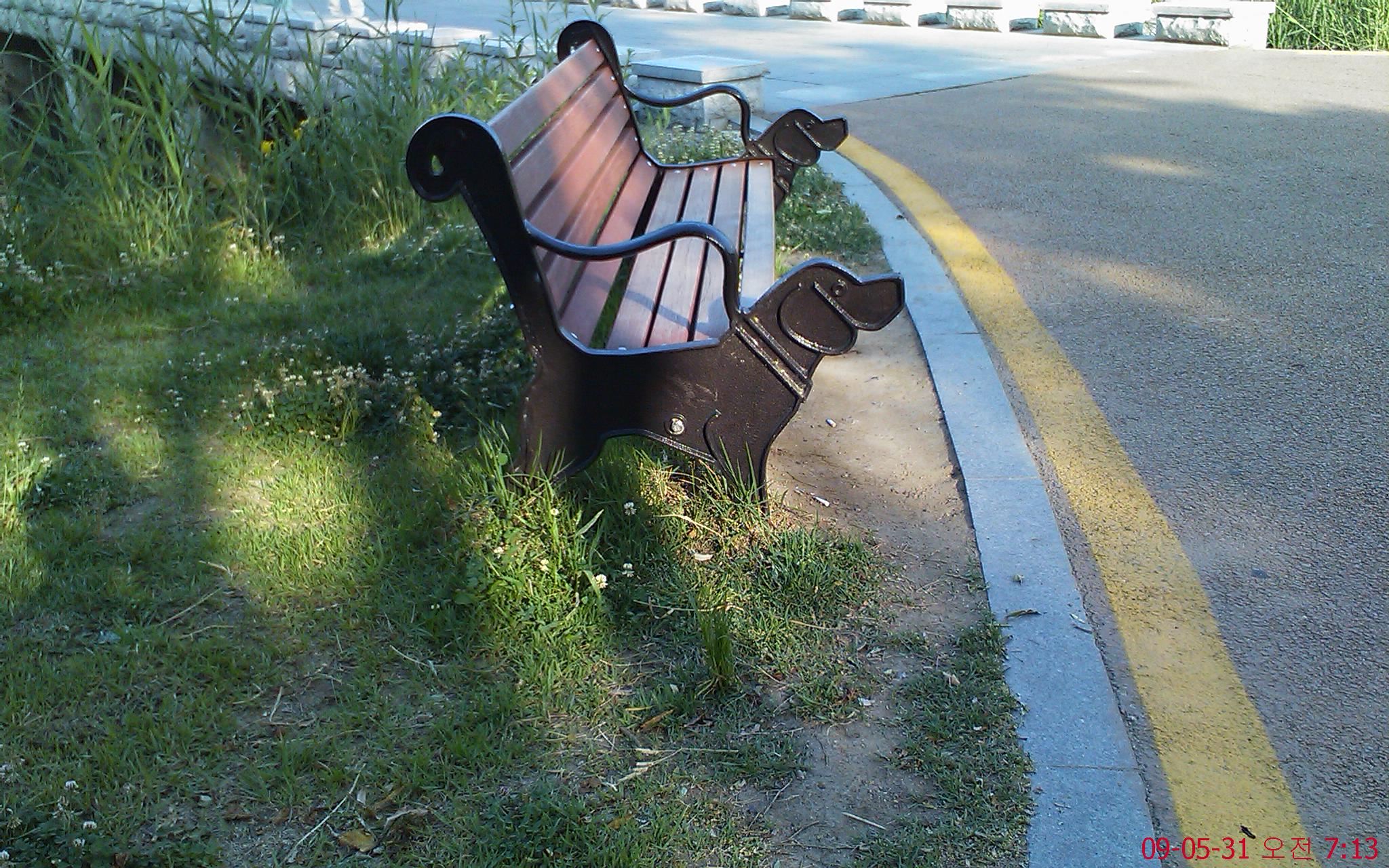This photograph captures a unique park bench situated along a roadway that transitions from pavement to concrete, with a yellow line and a white line along the road’s edge. The bench itself features brown wooden slats supported by black, wrought iron structures shaped like beagle dogs at each end. These dog-shaped supports have tails that wrap around to form the backrest, and their front and back legs serve as the legs of the bench. Notable details include the dogs' floppy ears, collars with silver rivets, and noses pointed skyward. The bench is positioned on a corner, with worn, light brown dirt in front, likely from frequent use. The surrounding area includes dark green grass dotted with clovers, tall light green plants with yellow and white flowers, and patches of dappled sunlight and shade, suggesting it’s mid-afternoon. A bridge with a low stone wall crosses the road further back, framed by tall grass and additional green plants. At the bottom of the image, the date “09-05-31” and some Chinese or Japanese characters are visible, along with the number “7-13.”